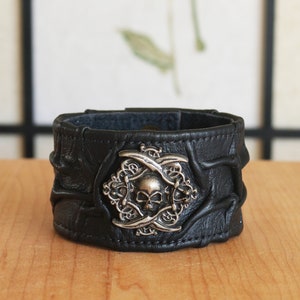This is a detailed photograph of a black leather wristband with a distinctive biker style. The wristband, which is slightly wrinkled to add texture and character, features a prominent silver skull emblem at its center. The skull is surrounded by ornate detailing, including scabbard-like embellishments on the top and bottom of the emblem, which sits on an interwoven metal piece that could be an octagon or diamond shape. The wristband is displayed upright on a light brown wooden table, reminiscent of a product showcase setup. The background features an out-of-focus white wall or possible Japanese-style screen, characterized by white panels bordered by black lines or bars.